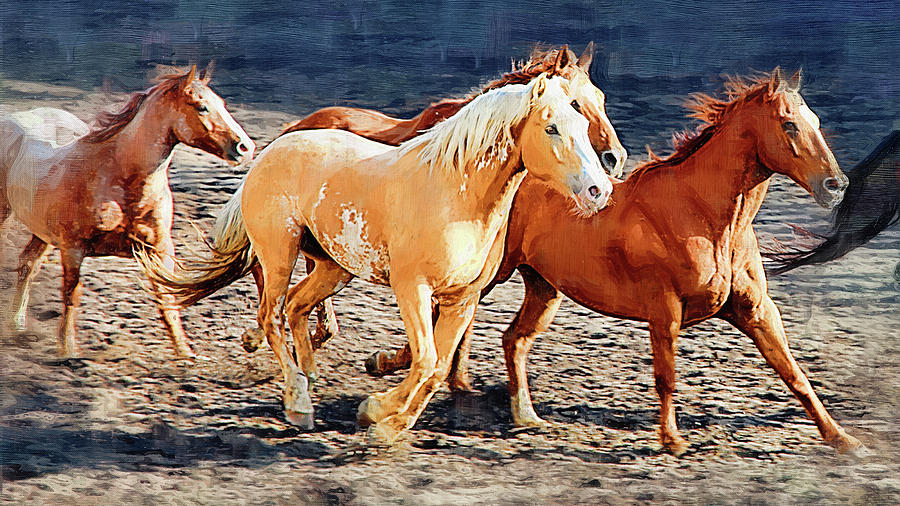The image depicts a stunning, photorealistic painting of a herd of wild horses galloping across a sandy beach. The horses, in various shades, are shown in dynamic motion, with some of their legs suspended mid-air, accentuating their gallop towards the right of the painting. At the forefront of the scene is a reddish-brown horse, followed closely by a distinctive tan horse with a blonde mane and white underbody. Further back, additional horses of similar reddish hues are visible. The background reveals dark water, suggesting the presence of an ocean or lake under the clear, sunny sky, as sunlight reflects off the horses' coats. The painter's masterful brushstrokes capture the fine details of the horses' eyes, bodies, and shadows, creating an intricate and captivating depiction of nature's raw beauty.